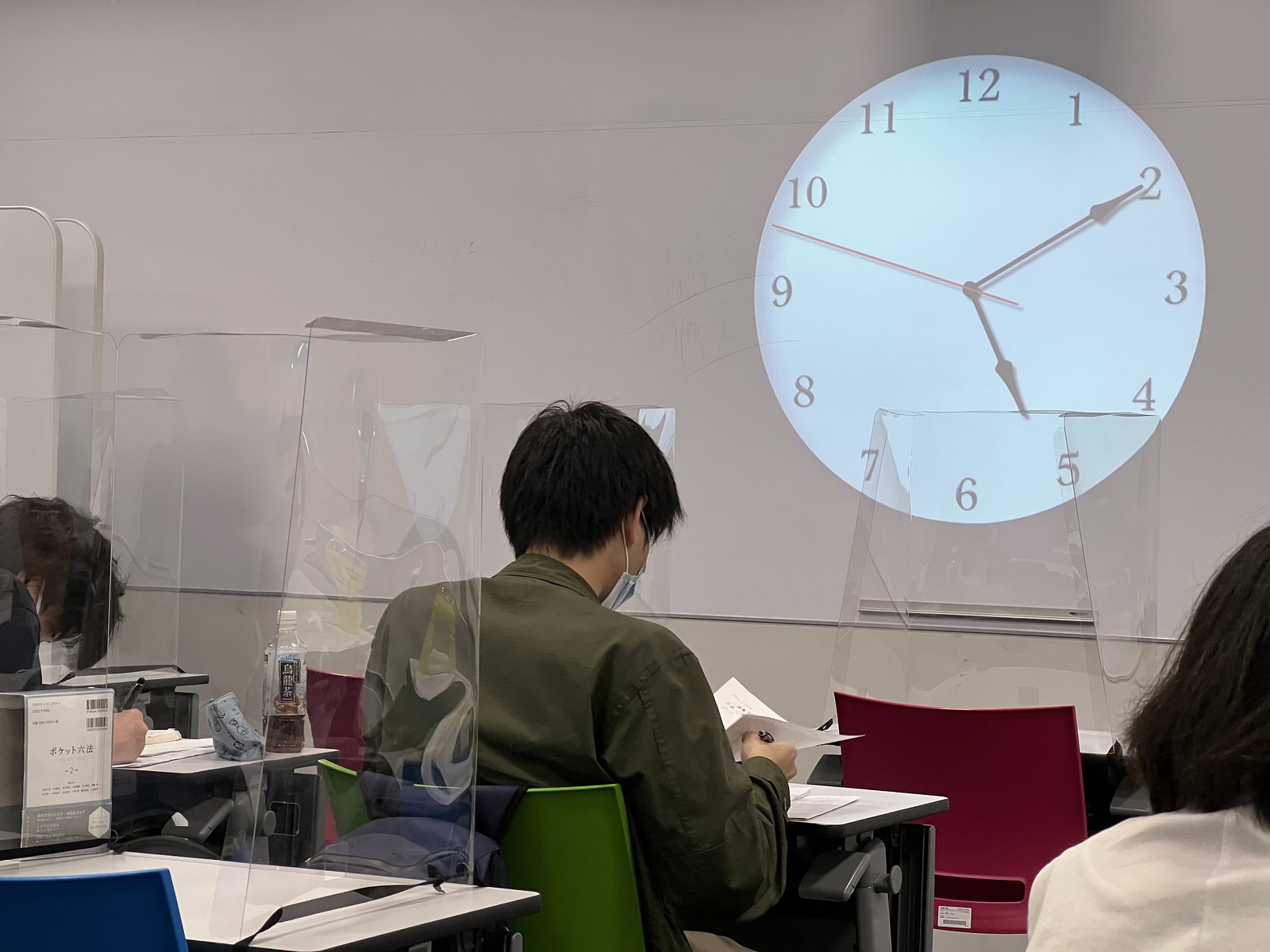This photograph captures a classroom setting with a significant wall clock displaying the time as 5:10. The clock features a white face and bold, dark numbers, prominently indicating the time. The image includes five desks, three of which are occupied by individuals with dark hair. These individuals, with their backs facing the camera, are seated at desks that are equipped with plexiglass barriers, likely installed for COVID-19 precautions. Two of the people are wearing masks; one is engrossed in writing on a piece of paper, while the other is holding and examining a document. The individual in the center, identifiable by his black hair and green shirt, is seated in a green chair. This detailed depiction highlights both the physical environment of the classroom and the activities of its occupants.